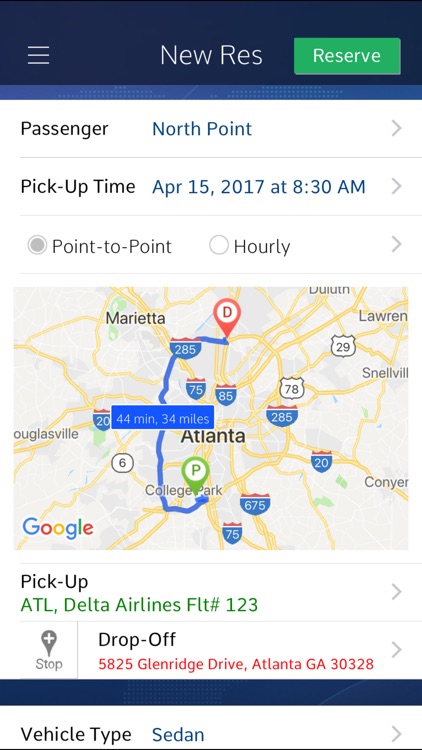This image is a screenshot of a navigation or booking app interface, likely related to transportation or a ride-hailing service. At the top of the screen, there's a prominent blue header bar that stretches horizontally across the display. Inside the center of this blue bar, written in white text, are the words "New Res." To the right of this text, there is a green button labeled "Reserve."

Directly below this main blue bar is a thinner blue bar. Beneath these bars, the main section of the window appears with various details. On the left side, it reads "Passenger," followed by "North Point." Below this, the text "Pick Up Time" indicates a scheduled time, which is April 15, 2017, at 8:30 AM. 

There are two options displayed side by side below the pickup information: "Point to Point" and "Hourly," with "Point to Point" being the selected option. Beneath these options, a map is shown displaying the travel route. Further down, the screen provides additional details about the pickup, stating "Pick Up Atlanta Delta Airlines Flight 123."